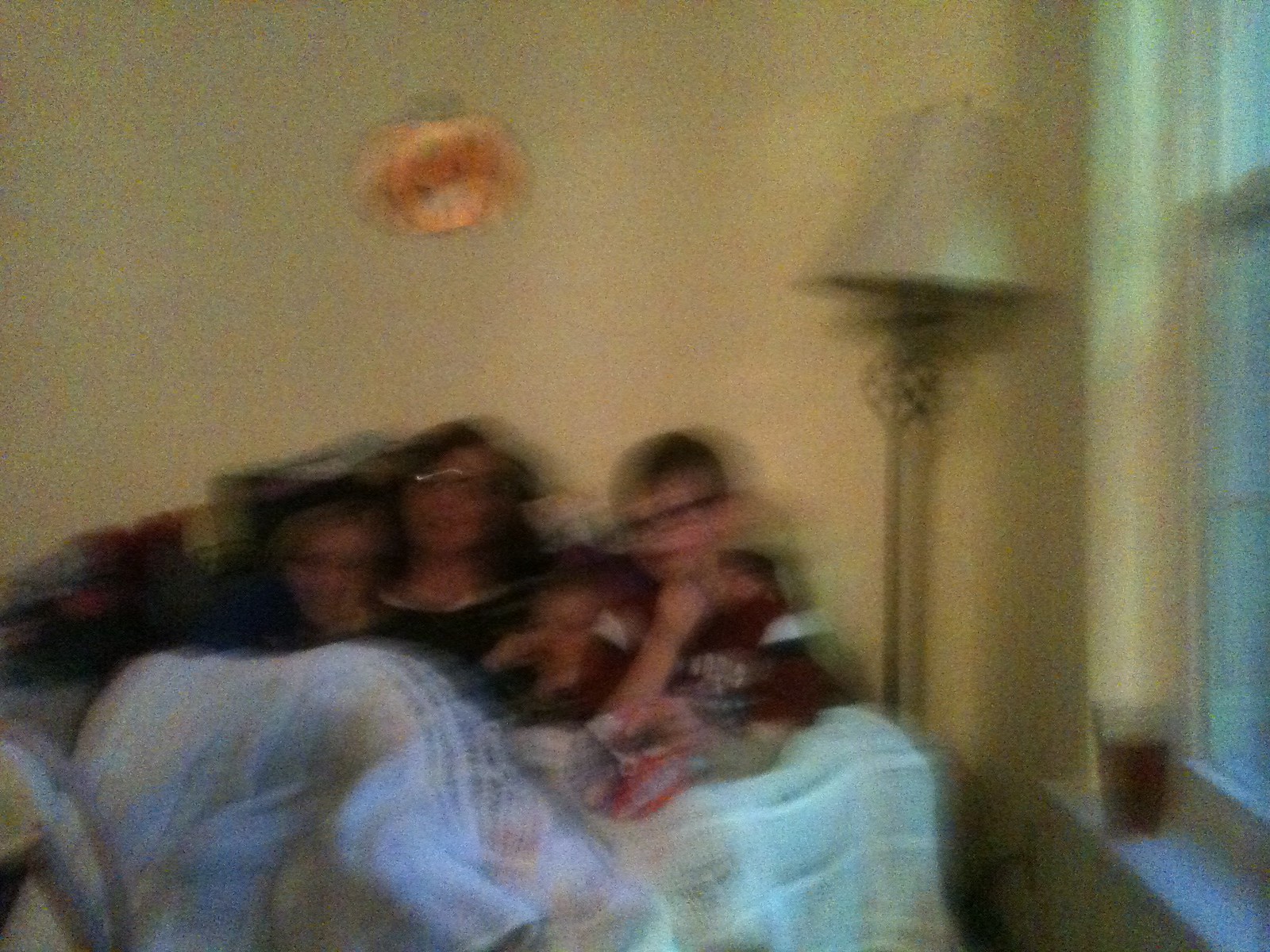In this dimly-lit, indoor photograph, a woman and three children, who all appear to be under the age of 11, are captured sitting closely together on a couch. Despite the shaky and fuzzy quality of the photo, the warmth and closeness of the family are evident. They are snuggled under a blanket, suggesting a cozy and intimate moment. In the background, a cartoon-like cutout of a jack-o-lantern hangs on the wall, hinting that it is fall or the Halloween season. To the side of the family, a floor lamp with a crooked shade casts a gentle glow, and on a nearby windowsill, there is a glass containing a brown drink. The scene portrays a comfortable, homey atmosphere filled with familial warmth and seasonal charm.